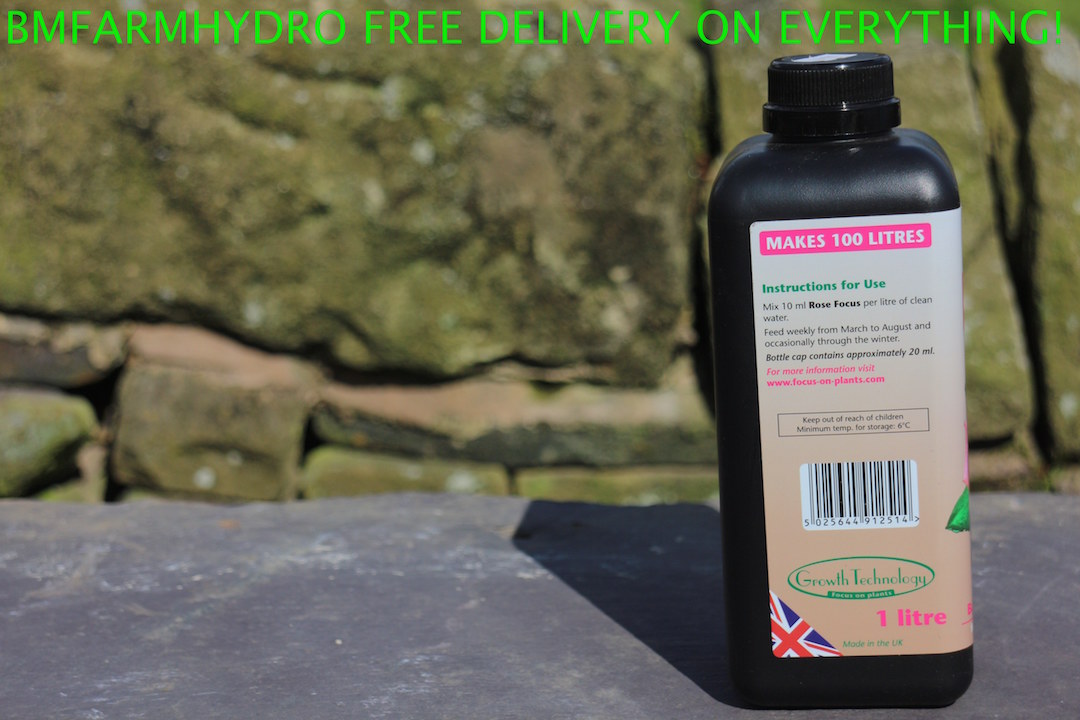This detailed landscape-oriented color photograph depicts a black plastic bottle of liquid plant food, prominently placed on the right-hand side of the image. The bottle, which has a black cap, occupies a significant portion of the frame, standing out against the outdoor setting. The surface beneath the bottle is a gray rock, while the background reveals a stone wall, emphasizing its natural setting.

Across the top of the image, in bright green text, the headline reads, "BM Farm Hydro, free delivery on everything!" This promotional message hints at a larger advertisement context for the photograph. 

The label on the bottle immediately catches the eye with a pink strip containing white text that states, "Makes 100 liters." Detailed instructions follow, indicating, "Instructions for use: Mix 10 milliliters of Rose Focus per liter of clean water. Feed weekly from March to August and occasionally through the winter. Bottle cap contains approximately 20 milliliters." Additional information advises, "Keep out of reach of children. Minimum temp for storage, 6 degrees Celsius," and directs viewers to visit "www.focusonplants.com" for more details.

The product label also includes "Growth Technology" in an oval logo and a partially visible Union Jack flag, signifying that the product is made in the UK. This image, with its emphasis on the product and clear instructive elements, serves as a comprehensive representation of plant food suitable for rose care.